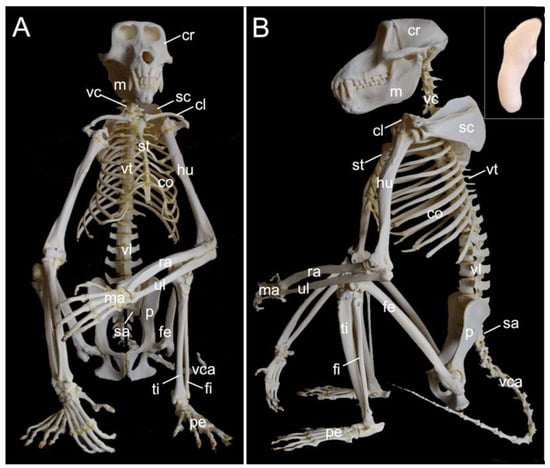The image features two highly detailed photographs of monkey skeletons, each labeled as "A" and "B" against a black background. 

Photo A, on the left, presents a frontal view of a white monkey skeleton. The skeleton is captured sitting on its hindquarters with its feet in front. Its left arm is slightly bent and resting on its knee, while the right arm hangs down in front of its leg. The skeleton's clavicle, skull, and other specific bone areas are annotated with letters such as CRSCCL.

Photo B, on the right, shows a side view of the same monkey skeleton, illustrating a profile where the nose points left and the back curves right. The skeleton maintains a similar seated posture, but this angle reveals its tail curving underneath it. The bones in this image are also marked with various letters. At the top right corner of this photo, there is a close-up insert, displaying a detailed section of the skeleton, which appears pinkish and whitish. Both images emphasize the intricate bone structure and annotations for further study or identification.